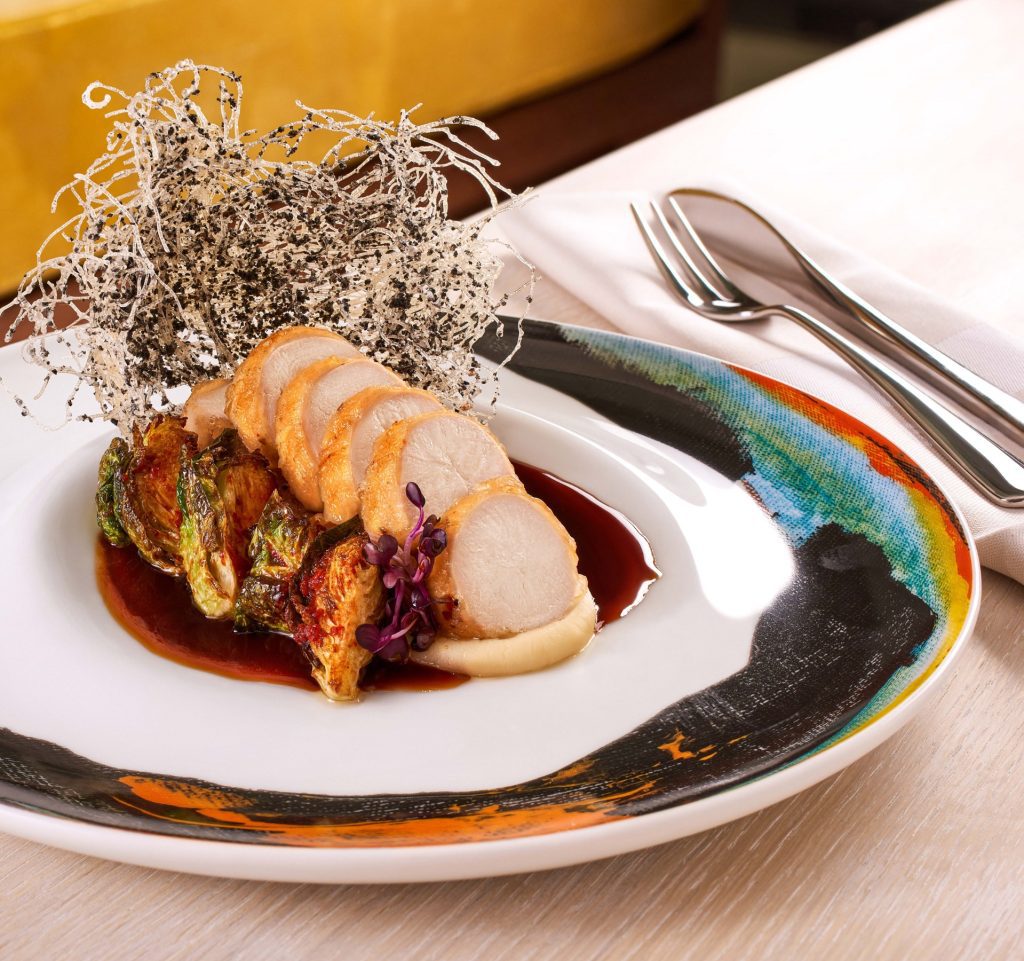In this detailed fine dining presentation, the centerpiece is a white plate adorned with an abstract, rainbow-colored pattern along its rim. At the heart of the dish, a rich, brown sauce—reminiscent of teriyaki—serves as the base. Elegantly arranged on top are six perfectly seared, quarter-sized chunks of what seems to be sliced pork loin, each piece featuring a soft white interior enveloped in a crisp, beige exterior. To the left, a cluster of oven-roasted Brussels sprouts nestles beneath the pork, partially soaked in the savory sauce. Adding a touch of sophistication, a delicate garnish of thin white strands speckled with black is draped elegantly behind the main elements. This artistic composition is placed on a light wooden table, accompanied by a neatly folded white napkin holding a polished silver fork and knife. The blurred golden-brown background hints at the upscale ambiance of this high-end restaurant.